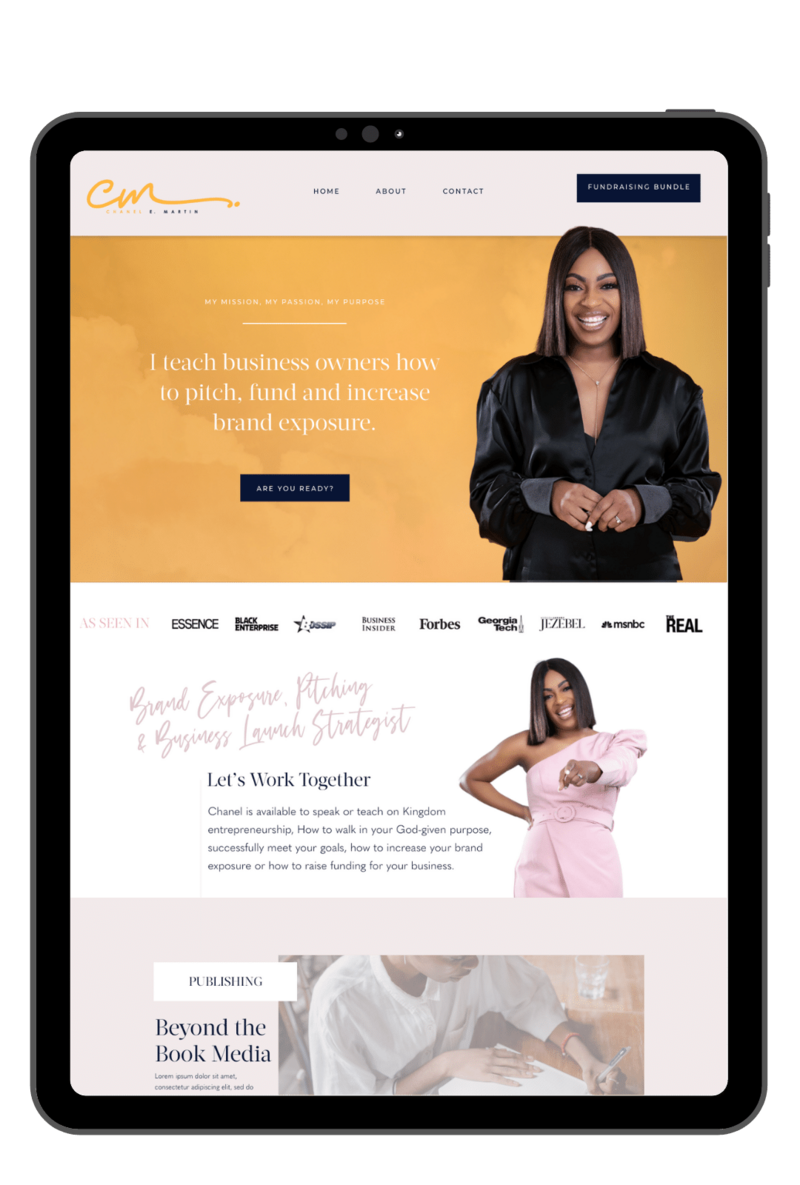The image showcases a tablet screen with a black border and a white header at the top, featuring a logo that merges the letters "C" and "M" in orange. There are three clickable areas within this header. To the right, there's a prominent black rectangle. Below this header, an orange section reads, "I teach business owners how to pitch, fund, and increase brand exposure," accompanied by an image of a woman dressed in a black shirt.

Directly underneath this orange segment is an area with a white background displaying several company logos, albeit too small and blurry to be identified. Adjacent to the logos stands an individual wearing a pink shirt, next to a text prompt, "Let's work together," followed by a descriptive paragraph. Further down, there is a section titled "Be on the Book Media," featuring an image of a person seemingly engaged in writing.